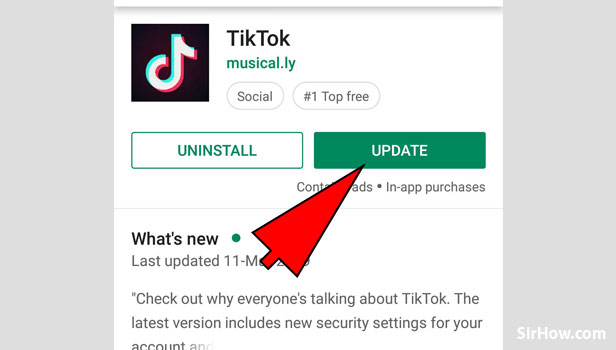A cropped screenshot captures a user in the Google Play Store, poised to update the TikTok app. The interface prominently displays the “Uninstall” and “Update” buttons, with a red arrow overlaid next to the latter, indicating their intention to perform an update. The screen includes various details such as a “What's New” section highlighting the app's latest security updates and features, and promotional text encouraging users to discover why TikTok is making waves. Additional tags categorize the app under "social," "number one," and "top free," and descriptors mention in-app purchases. The background of the interface is white, with black text, and the TikTok logo is visible. Interestingly, the URL listed is musical.ly, referencing the app's former brand. The bottom right corner of the screenshot bears a watermark from “sirhow.com.” The shot effectively illustrates the process of updating the TikTok app on the Google Play Store.